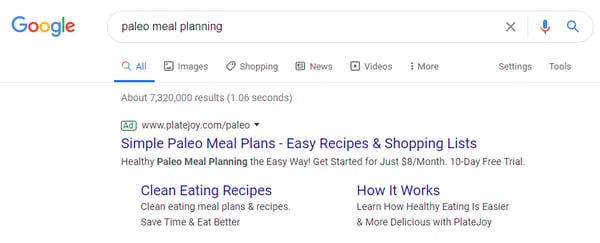This screenshot captures a desktop application featuring the Google homepage. In the top left corner, the iconic Google logo is prominently displayed. In the search bar, the query "Paleo meal planning" is entered, accompanied by an 'X' button on the right for clearing the search. Adjacent to the 'X' are a microphone icon and a magnifying glass, indicating options for voice search and initiating the search, respectively.

The highlighted tab below the search bar indicates the 'All' results category, with other tab options including 'Images,' 'Shopping,' 'News,' 'Videos,' and 'More' arranged to the right. The area below these tabs displays toolbar options labeled 'Settings' and 'Tools.' The results section starts with a note indicating that approximately 7,320,000 results were found within 1.06 seconds.

The first result is an advertisement by PlateJoy, denoted by the URL www.flatejoy.com with a dropdown arrow for more options. The ad promotes simple Paleo meal plans, boasting easy recipes and shopping lists aimed at making healthy Paleo eating straightforward and affordable. The offer includes a $8 per month plan with a 10-day free trial period.

Beneath this, there is a link titled "Clean Eating Recipes," which highlights clean eating meal plans and recipes designed to save time and improve nutrition. Adjacent to this is another link titled "How It Works," encouraging users to discover how PlateJoy can make healthy eating both easier and more delicious.

The entire content appears on a predominantly white background, ensuring a clean and uncluttered user interface.